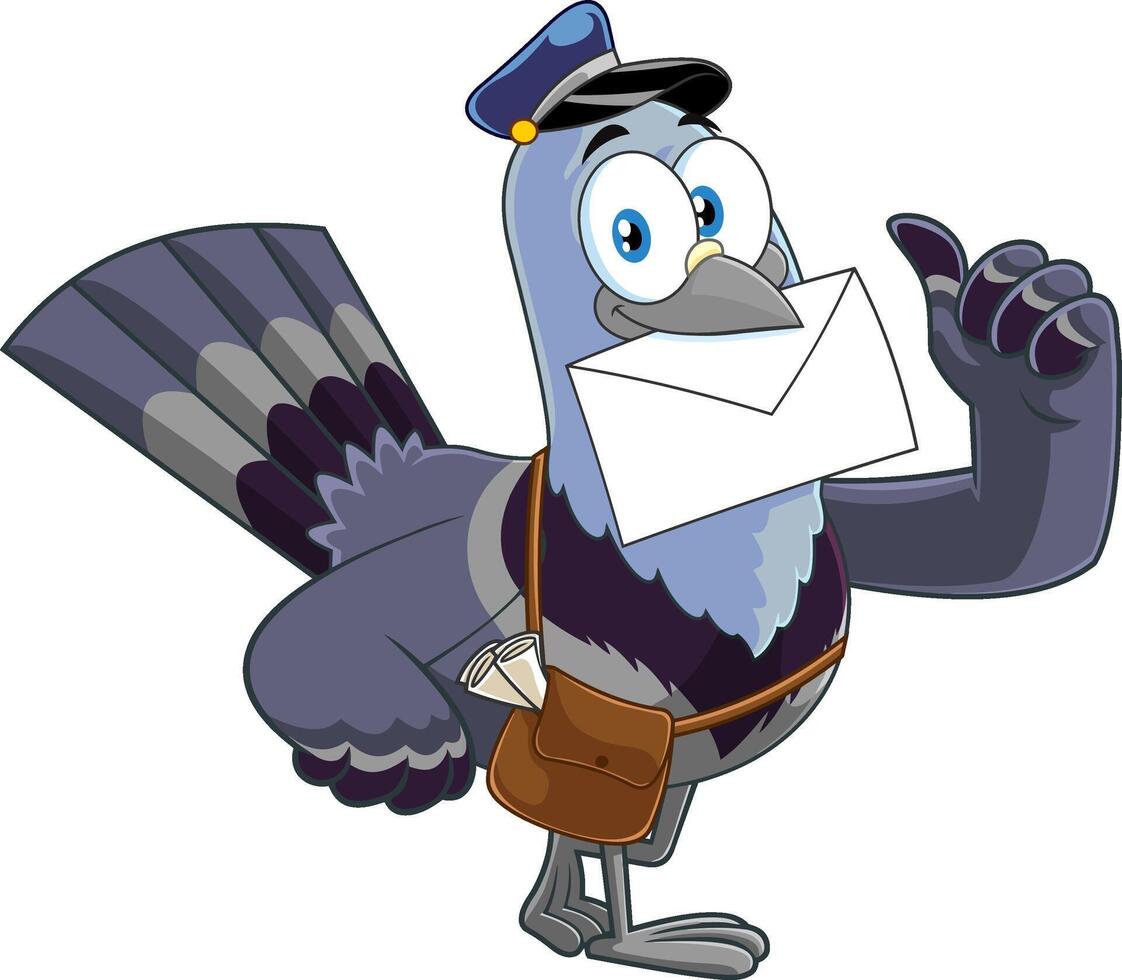A cheerful bird, resembling a postal carrier, is depicted in vibrant shades of blue, gray, and dark blue, mirroring the uniform colors of the U.S. Postal Service. The bird wears a traditional postal hat and has striking blue eyes, accentuating its animated expression. With a letter held firmly in its beak, the bird gives a thumbs-up, exuding a positive and confident demeanor. A classic leather mail pouch is slung stylishly over one shoulder, resting across its chest feathers, as it struts with an air of self-assurance. The well-drawn cartoon scene suggests efficiency and readiness, hinting at the reliable services of the U.S. Postal Service, potentially alluding to the concept of air mail. The image effectively combines whimsical art with practical messaging, making it a strong candidate for an engaging advertisement.